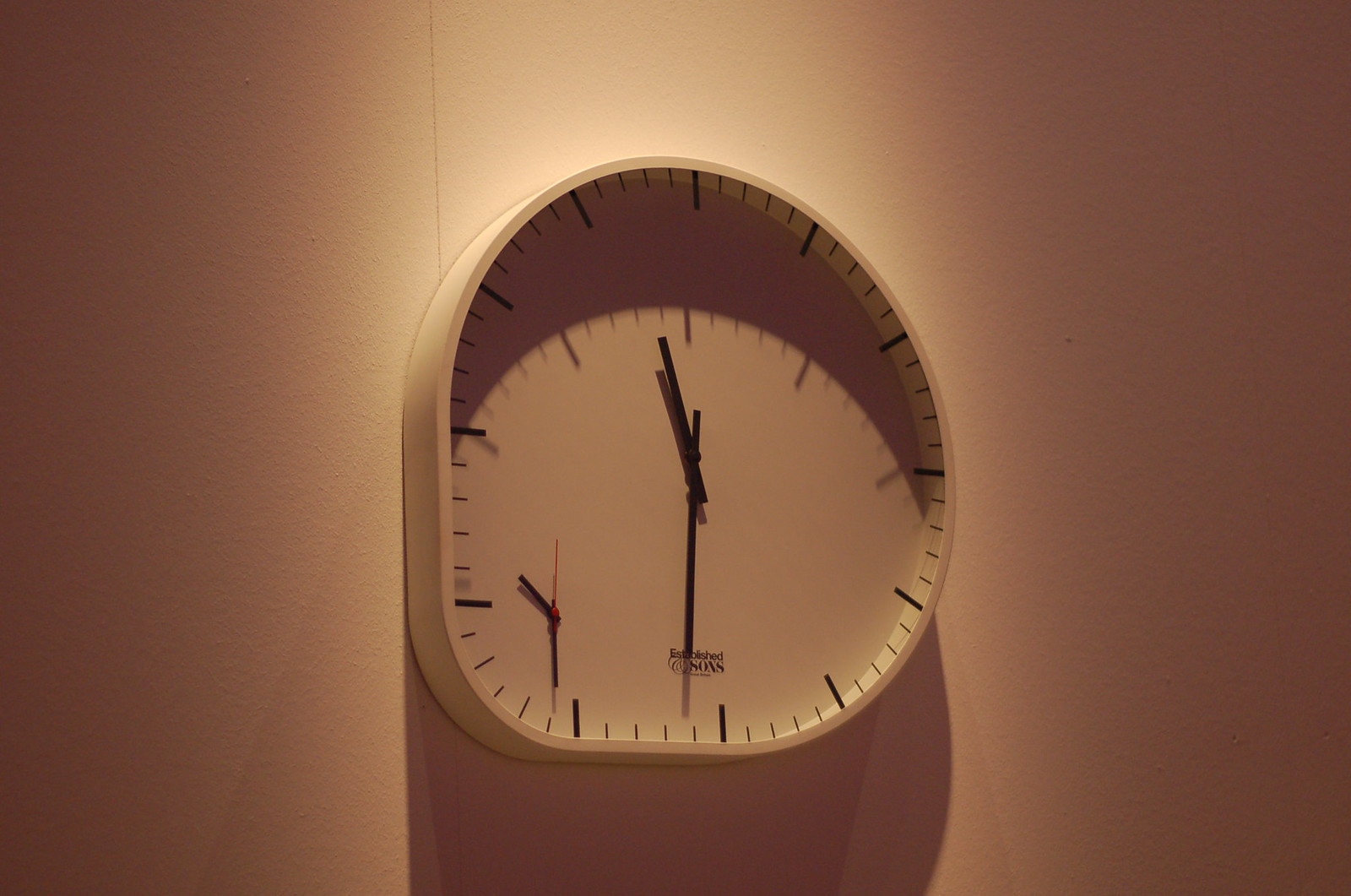In this image, we see a white wall adorned with an unusual and intricate clock. The clock's design is asymmetrical; it primarily retains a circular shape on the top and right sides, but the bottom side is flat before curving gently into the left side. The left side of the clock is particularly unique, resembling an elbow rather than completing a perfect circle.

The clock face is minimalistic, lacking numerical indicators but marked with minimalist lines to denote where the numbers 1 through 12 would typically be. It features two sets of hands. The central section houses the traditional hour and minute hands, while an additional, smaller clock is positioned in the bottom left corner, complete with hour, minute, and second hands. The second hand in this smaller section is distinctively red, providing a pop of color against the otherwise monochrome background.